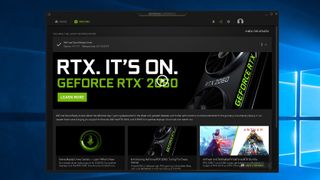This image is a screenshot of a website showcasing NVIDIA's GeForce RTX 2060 graphics card. At the top of the page, bold text displays "RTX. It’s On." The backdrop appears to feature graphics reminiscent of speaker outlines or abstract elements, creating a visually intriguing background. Prominently, the text "GEFORCE RTX 2060" runs across the image with a partially obscured play button overlapping the numbers, hinting at an embedded video. The background features a distinctive Windows interface with blue and teal Windows logos on the right, casting radiant lines across the scene. A prominent black rectangle overlays this backdrop, housing the primary content.

In the upper right corner of this rectangle, there's a clickable white headphone icon suggesting additional audio-related content or support. Below, a horizontally-aligned panel reiterates the "RTX. It’s On" slogan alongside "GeForce RTX" and "2060." Adjacent to this slogan is a "Learn More" button, inviting viewers to explore further details about the product. At the very bottom, three additional rectangular sections provide snippets of information, enhancing the webpage's layout and guiding users toward relevant insights.